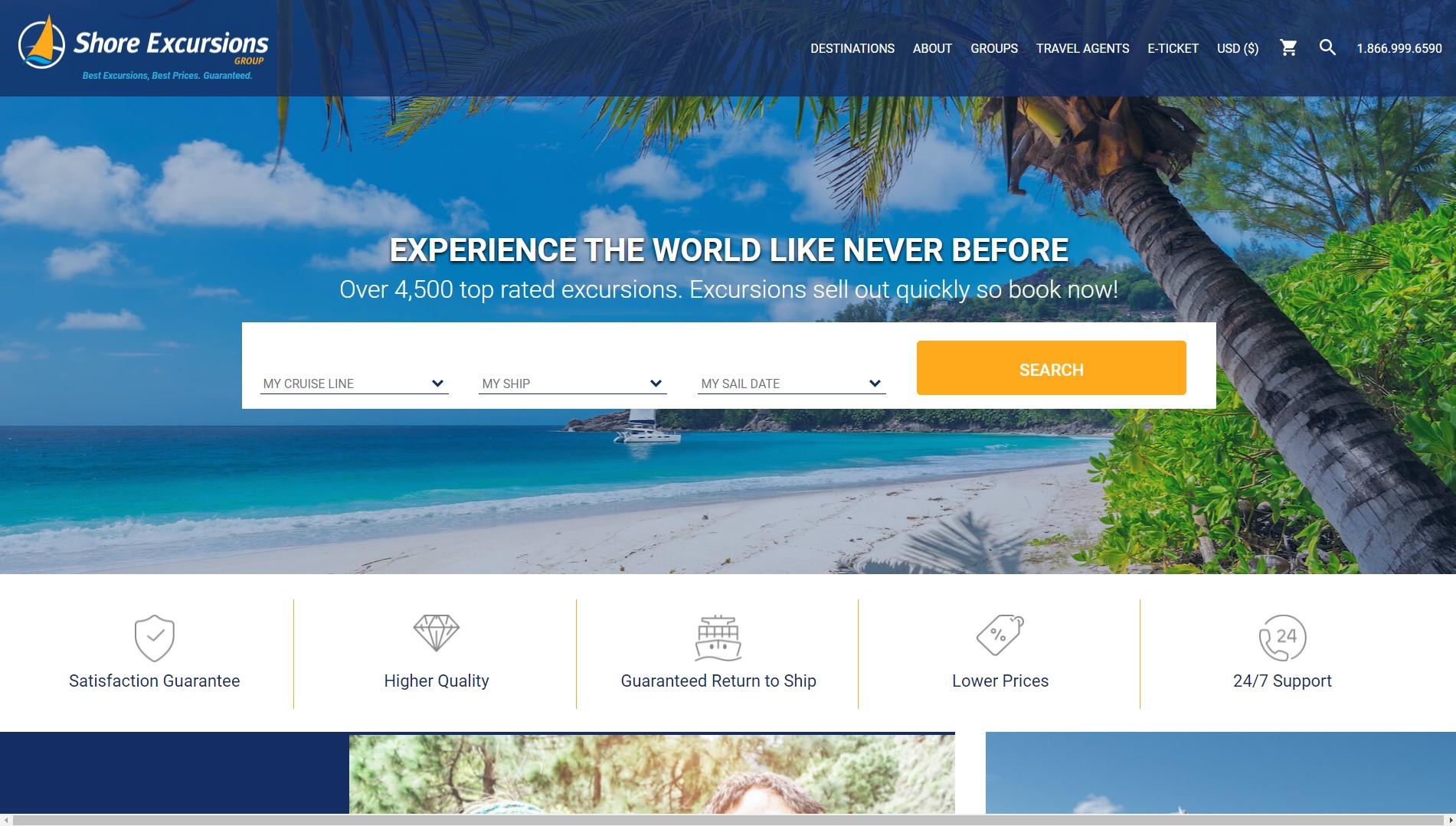The image showcases the homepage of the Shore Excursions Group website. On the left-hand side, prominently displayed, is the company name "Shore Excursions Group," accompanied by a silhouette of a sail within a white circle. Positioned along the same top bar is a horizontal menu in white font featuring the options: Destinations, About, Groups, Travel Agents, E-Ticket, USD, followed by icons for a shopping cart and a magnifying glass, and a contact phone number. This top bar is semi-transparent, allowing the background image to subtly show through.

The background image is a picturesque scene of a beach with a pristine backdrop of a palm tree and a small sailboat. The palm tree elegantly enters the frame from the bottom right-hand corner, lending a tropical flair.

Centrally located within the image is a search bar, framed by the tagline "Experience a World Like Never Before" at the top. Just beneath this inspiring motto, the website declares, “Over 4,500 Top-Ranked Excursions. Excursions Sell Out Quickly, so Book Now.” Directly below this call to action is the search bar, providing options for selecting 'My Cruise Line,' 'My Ship,' and 'My Sail Date,’ encouraging users to find and book their ideal excursions.